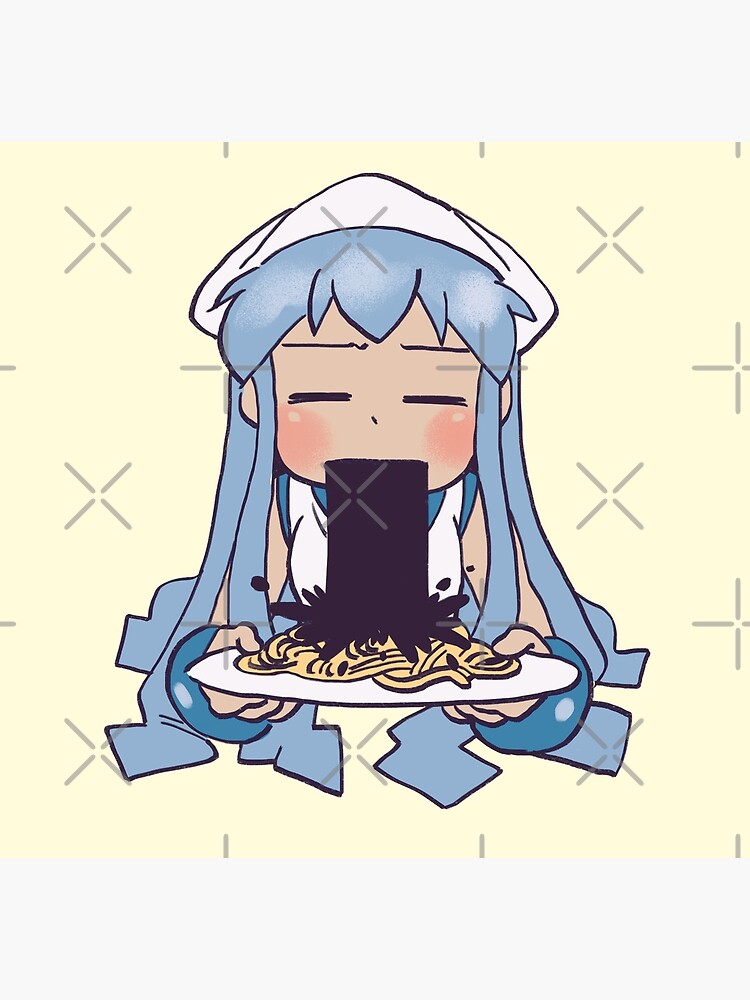The image is a cartoon anime-style drawing featuring a girl with long, light blue hair that flows down to the floor. She is seated and holding a white plate filled with orange or yellow spaghetti. The girl, who has her eyes closed depicted as simple lines, is wearing a white, nurse-like hat and a sleeveless top that is a mix of white and blue. She's shown vomiting a pitch-black liquid onto the spaghetti, with the liquid emerging from her mouth in a straight rectangle before splashing onto the plate and spreading out. The background is yellow, adorned with repeated X-shaped watermarks and stars, giving texture to the scene. Only the upper part of her body and her knees are visible in the image.